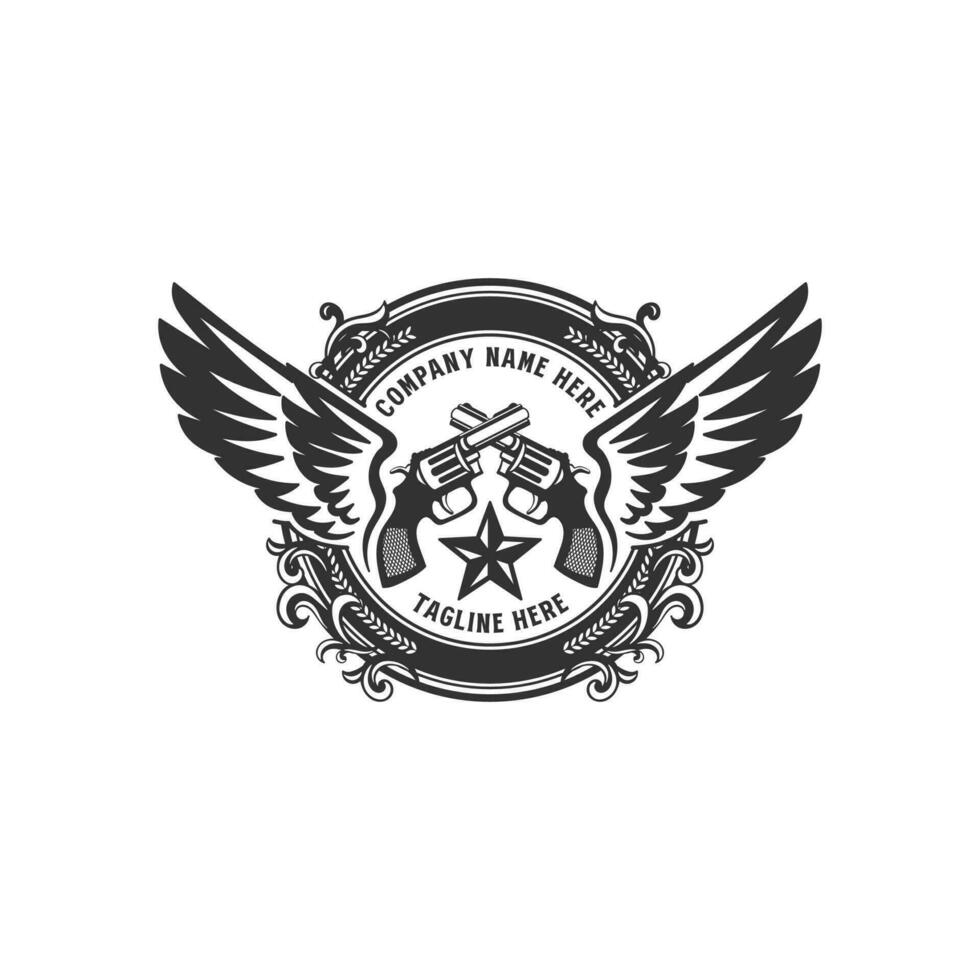This black and white illustration presents a vintage-inspired circular logo featuring symmetrical, intricate designs. At the center of the logo, two crossed handguns form an X, with a star positioned below them. Adjacent to the pistols, a pair of eagle wings with two layers of feathers extend outward, adding a sense of grandeur and balance. Surrounding the central elements is a prominent black circle, bordered by smaller black and white circles, and adorned with elegant floral and ornamental motifs that mirror each other on either side. The top of the circle showcases the placeholder text "company name here" in a semicircle, while the bottom includes the text "tagline here." The entire composition is rendered in a detailed, black-and-white cartoon style, giving it a retro, yet sophisticated appearance.